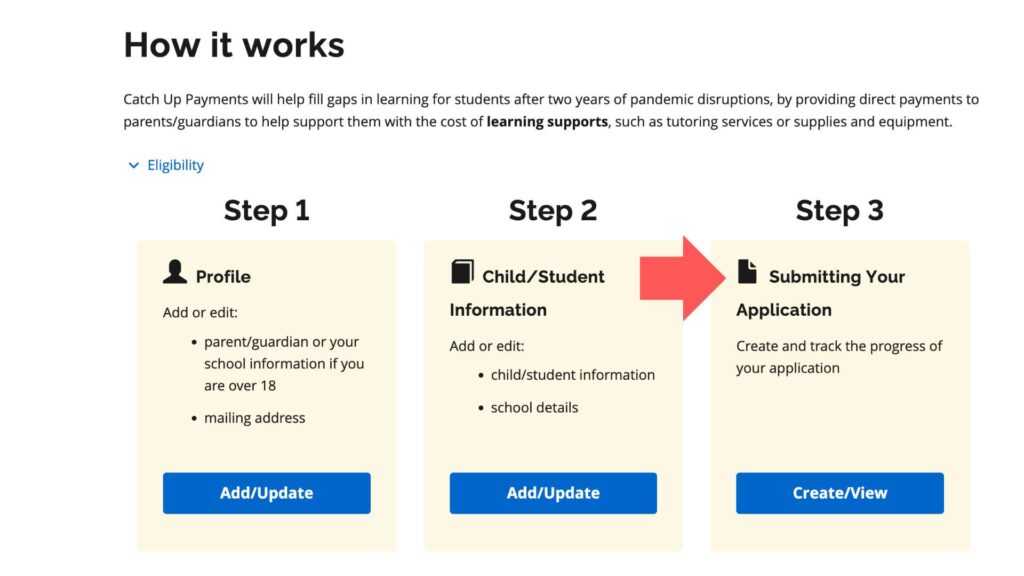The image depicts a website with an informational section outlining a three-step process for accessing catch-up payments aimed at addressing learning gaps caused by two years of pandemic disruptions. Dominated by the large, bold heading "How It Works," the page explains that direct payments will be made to parents and guardians to help cover the costs of learning support, including tutoring services and necessary supplies or equipment.

### Step-by-Step Breakdown:
1. **Step One: Profile Information**
   - **Description**: Users can add or edit profile information, including details for parents or guardians. This step also accommodates users over 18, allowing them to input their school information and mailing address.
   - **Button**: A blue "Add/Update" button facilitates these changes.

2. **Step Two: Child Student Information**
   - **Description**: This section requires users to add or update information regarding the child student and their school details.
   - **Button**: A blue "Add/Update" button is also present here.

3. **Step Three: Submitting Your Application**
   - **Description**: Users can create and track the progress of their application in this final step.
   - **Button**: A blue "Create and View" button is available for this action.
   - **Visual**: A thick red arrow directs from Step Two to the "Create and View" box in Step Three, indicating the progression to the final step.

The background of the website is entirely white, and while the steps themselves are clear, no additional conclusions or next steps are provided beyond Step Three.